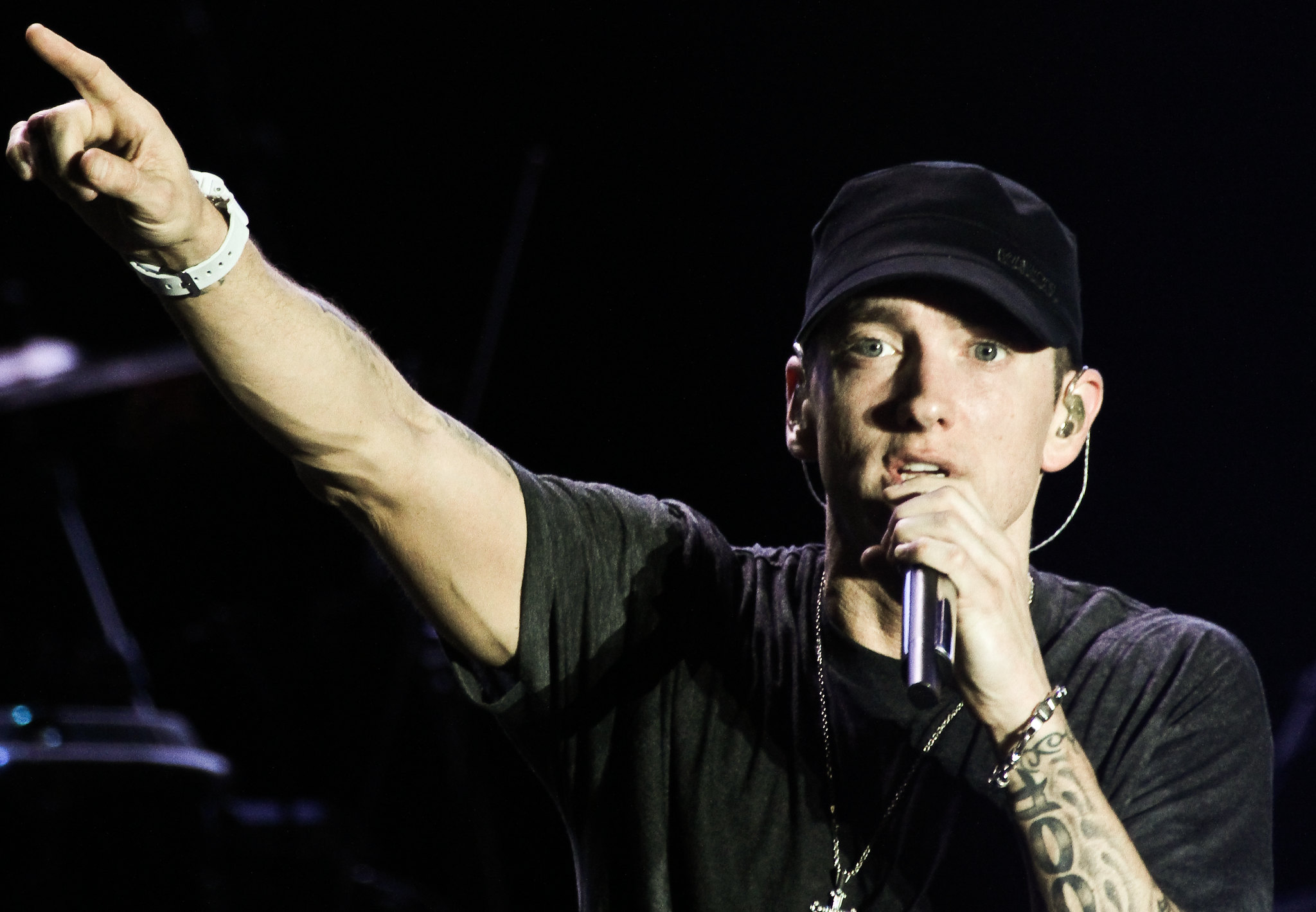This is a photograph of rapper Eminem performing on stage. He is wearing a black short-sleeved t-shirt, a black cap, and a silver chain necklace with a cross pendant. Eminem's left wrist is adorned with a metal bracelet, and his tattooed forearm is clearly visible. On his right wrist, he sports a white watch, and he is holding a microphone up to his mouth with one hand while pointing into the audience with his other hand. He has earpieces fitted around both ears, with wires running behind his neck. The background is predominantly black with some performing equipment partially visible on the left side. The image captures a youthful Eminem in what appears to be a dynamic and energetic moment on stage.